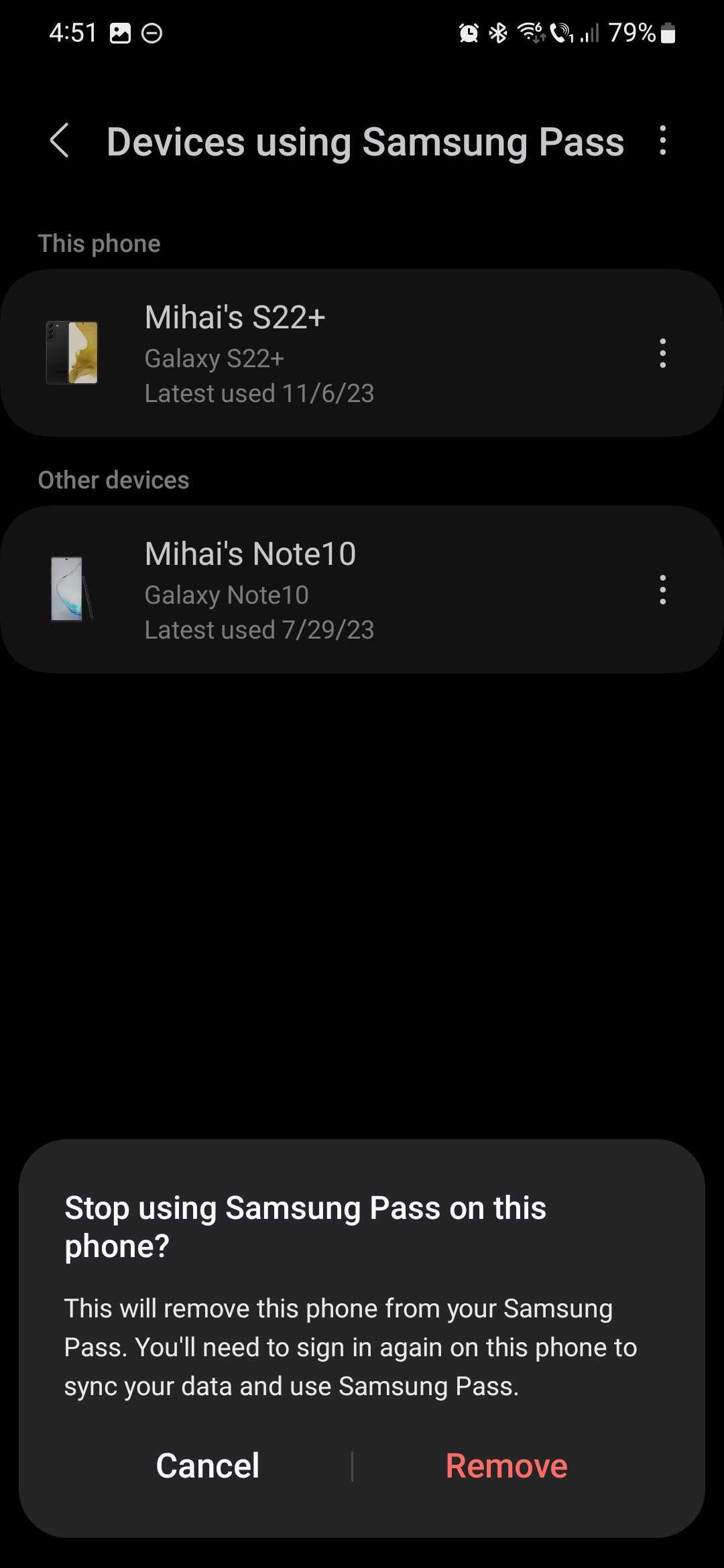Screenshot from a mobile phone in dark mode with a black background. The time is displayed in the upper left corner, reading 4:51 in white font. To the right are various icons, including a photo icon, a small circle with a dash, an alarm clock icon, a Bluetooth icon, a Wi-Fi signal icon, a Wi-Fi calling icon, and a mobile signal icon. The text "79%" is shown next to a battery icon. 

Below this status bar, a white font line reads "Devices using Samsung Pass." To its left is a back arrow, and to the right are three vertical white dots. Underneath, in gray font, it says "This phone." A gray rectangle below this contains white text that reads "Mihai's S22+", followed by gray text stating "Galaxy S22+. Latest used, 11/6/23." An illustration of a Galaxy S22+ is placed to the right.

Further down, against a black background, gray text reads "Other devices." Another gray rectangle lists "Mihai's Note 10," followed by "Galaxy Note 10" in white font.